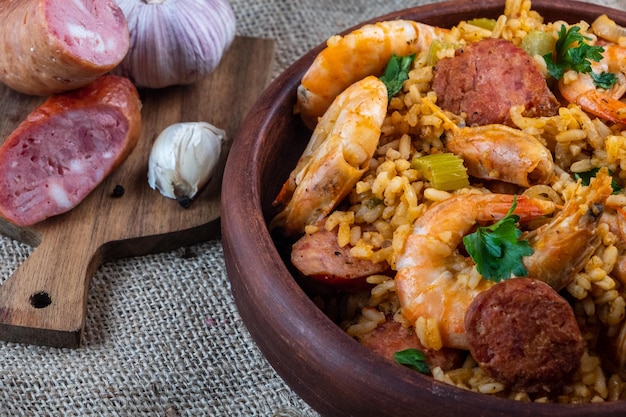The image vividly captures a close-up view of a vibrant meal setting. On the right, there is a substantial dark brown wooden bowl filled almost to the brim with a hearty shrimp and rice dish, akin to a jambalaya. The rice has a rich, yellow-orange hue interspersed with plump shrimp that still have their heads and tails intact, adding an authentic, rustic touch. Mixed within are slices of brownish-red sausage, possibly andouille, and sprigs of fresh herbs like cilantro or parsley, enhancing the dish's visual and aromatic appeal. 

On the left side, there is a small brown wooden cutting board, shaped like a pan, which holds two reddish-brown sausage links placed at different angles. Accompanying the sausages are two garlic heads—one fully intact and another partially peeled—adding a rustic charm to the presentation. The scene is set on a gray burlap cloth, providing a textured, earthy background that complements the rich colors of the food. The lighting is bright and clear, showcasing the detailed textures and vibrant colors in the image.